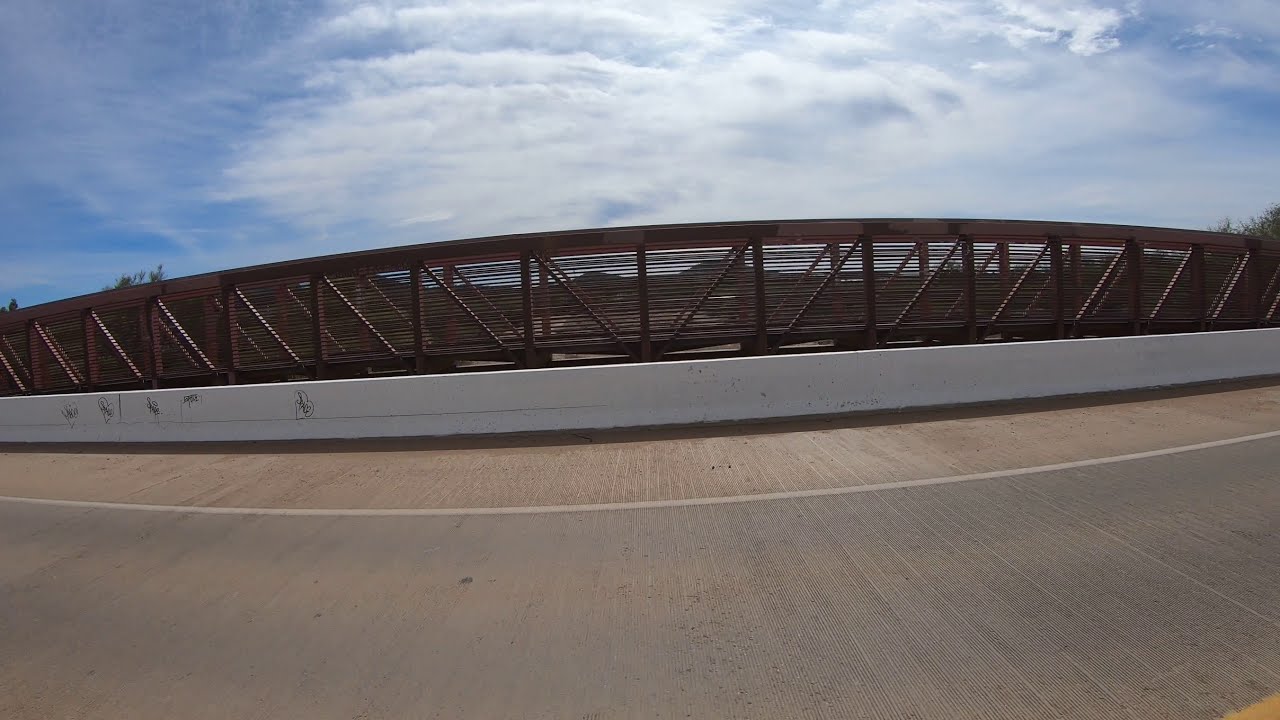This horizontal rectangular image captures a section of a modern roadway, potentially a bridge, adorned with a smooth, pinkish-tan concrete surface and a faint yellow center line visible at the bottom right corner. The road is flanked by a half-foot high, white barrier wall, topped with a slightly arch-shaped brown railing, indicating a pedestrian walkway alongside it. This walkway is securely enclosed with a mesh, preventing access from the walkway onto the roadway or the other side. The empty road spans the foreground with no visible vehicles or people, conveying a sense of quietness. A vibrant blue sky with light, scattered clouds towers above, setting a crisp contrast against the earth tones of the bridge. In the distance to the right, treetops and faint silhouettes of hills hint at a natural landscape beyond. The scene's primary colors—brown, blue, and white—create a serene and somewhat scenic atmosphere, giving the impression of a well-maintained, newly constructed passage.